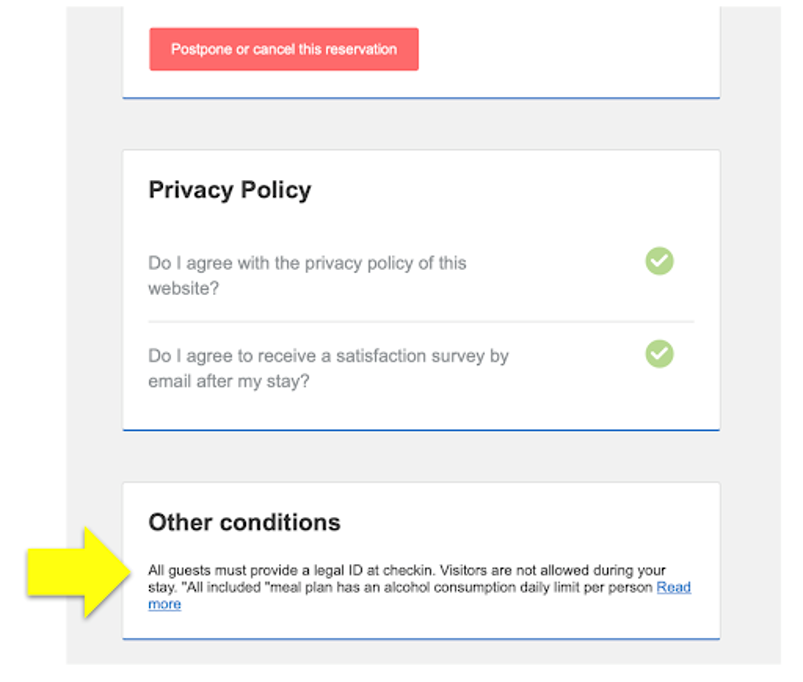The image is a close-up of a screen displaying various sections related to a reservation. At the very top, there is clear white text set against a red background that states "Postpone or cancel this reservation." Below this, a blue line separates the header from the rest of the content, which is displayed against a light gray background divided into horizontal sections.

The first section features the text "Privacy Policy," followed by two questions. The first question asks, "Do I agree with the privacy policy of this website?" with a green check mark indicating agreement displayed to the right. The second question is, "Do I agree to receive a satisfaction survey by email after my stay?" which also has a check mark next to it, signifying agreement.

The next section outlines "Other Conditions" and includes several stipulations:
- All guests must provide a legal ID at check-in.
- Visitors are not allowed during the stay.
- The all-inclusive meal plan has a daily alcohol consumption limit per person.

At the end of this section, there is a "Read more" link in blue text. To the left of this final message, a yellow arrow points to the right. The light gray background continues to be the default wherever there is no text or other elements displayed.